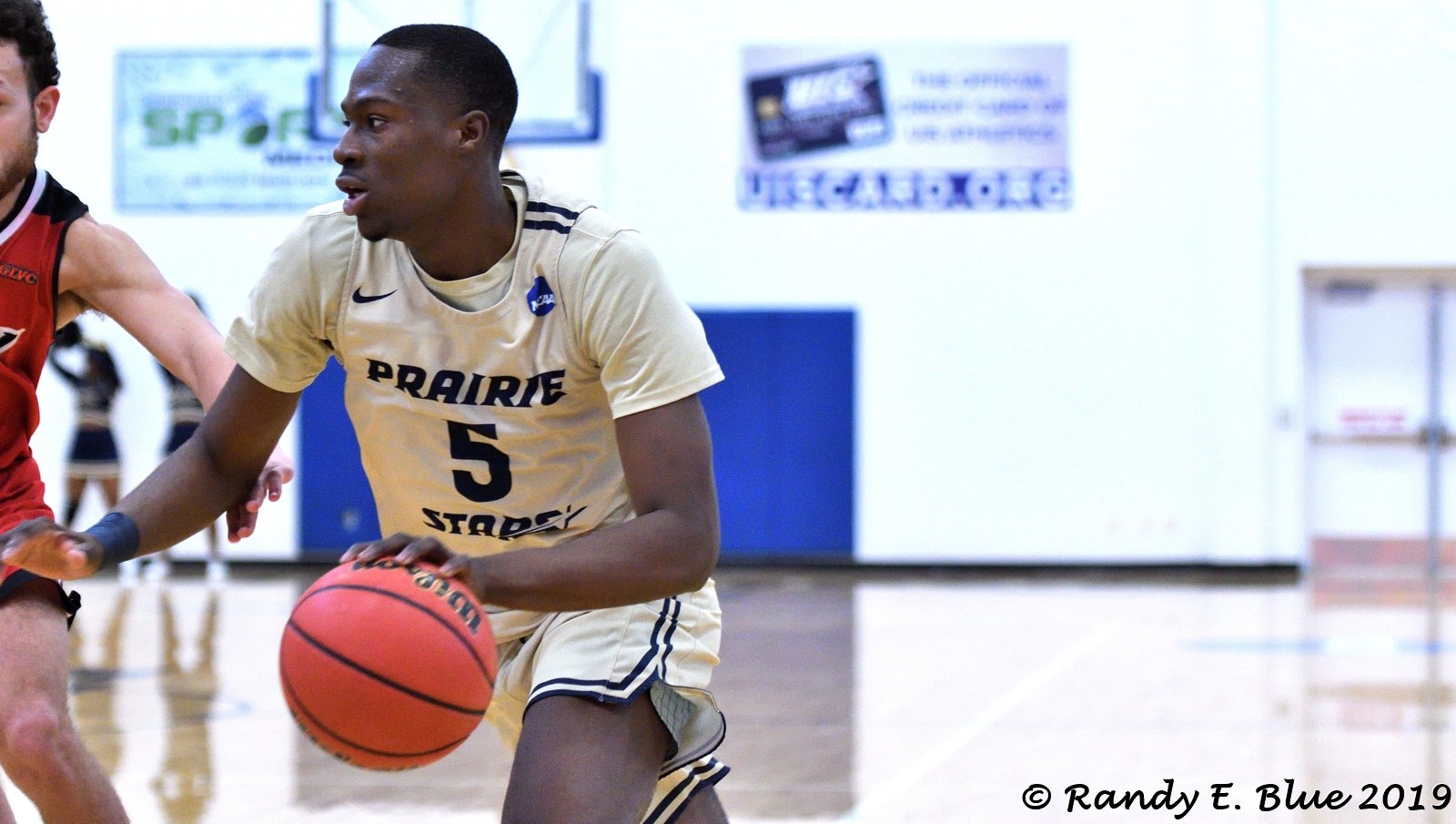The image captures a high-energy moment from a basketball game inside a gymnasium. Central to the action is a black teenager, the main character, dribbling a basketball with his left hand as he advances towards the basket. He is donned in a primarily white jersey with blue trim, bearing the inscription 'Prairie Stars' and the number 5. Underneath his jersey, he wears a white t-shirt. His gaze is focused intently to his left. Partially visible in the frame is his opponent, who is wearing a red uniform, hinting at an ongoing defensive play. The backdrop of the photograph reveals the setting in more detail: white walls with blue accents, a hardwood basketball court, a glass door on the right, and what looks like a poster and backboard. Cheerleaders can be seen practicing in the blurry background on the left side. All these elements come together to depict a dynamic and engaging moment in a possibly high school or college basketball game.